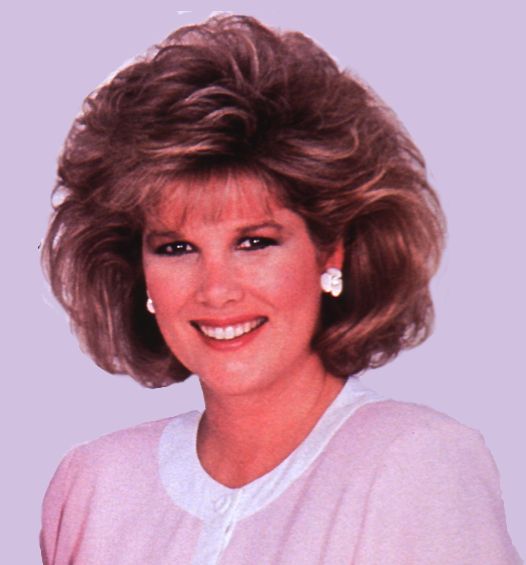This is an up-close, vintage image from the 1980s featuring a woman smiling directly at the camera. She has short, voluminous light brown hair that is teased and poofed up, with thin bangs in the front, exuding the characteristic hairstyle of the era. Her left ear is visible, adorned with white flower earrings. The background of the image is a light pink or light purplish color, possibly a studio setting. The woman wears a delicate white-collared shirt with a button at the top, where the collar and buttoned area are white, and the rest of the shirt is a very light pink. The image is cut off at the chest, showing only the top portion of her outfit. The woman is looking directly at the camera with a big smile, featuring noticeable red lipstick, enhancing her cheerful expression.